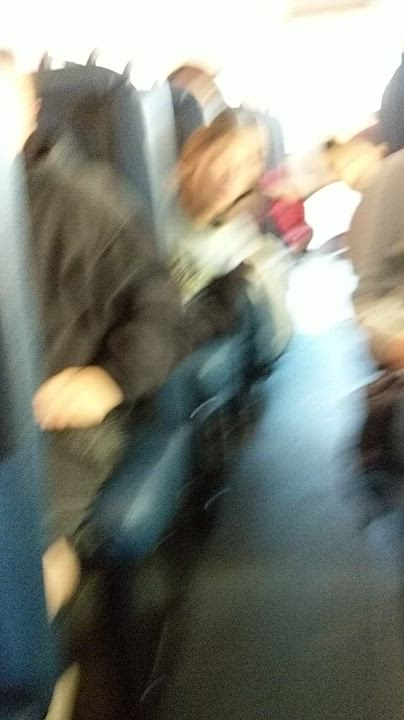This exceedingly blurry photograph appears to be taken in the aisle of a crowded bus. The image captures several indistinct figures, including a man on the left side, where only part of his head, hand, and dark jacket are visible. In front of him is a blue seat with a tall back, typical of bus seating arrangements. Behind him, a woman with long blondish hair, wearing a white shirt, is leaning into the aisle, seemingly looking directly at the camera. The aisle itself is a darkish teal gray, stretching toward the back where a very bright white light suggests the presence of an exit door. Further down the aisle, potentially another person can be seen across from the woman though the details are extremely unclear. The right side of the aisle remains very blurry and undefined, contributing a chaotic feel to the image. The overall slant of the scene seems to run from the southwest to northeast.